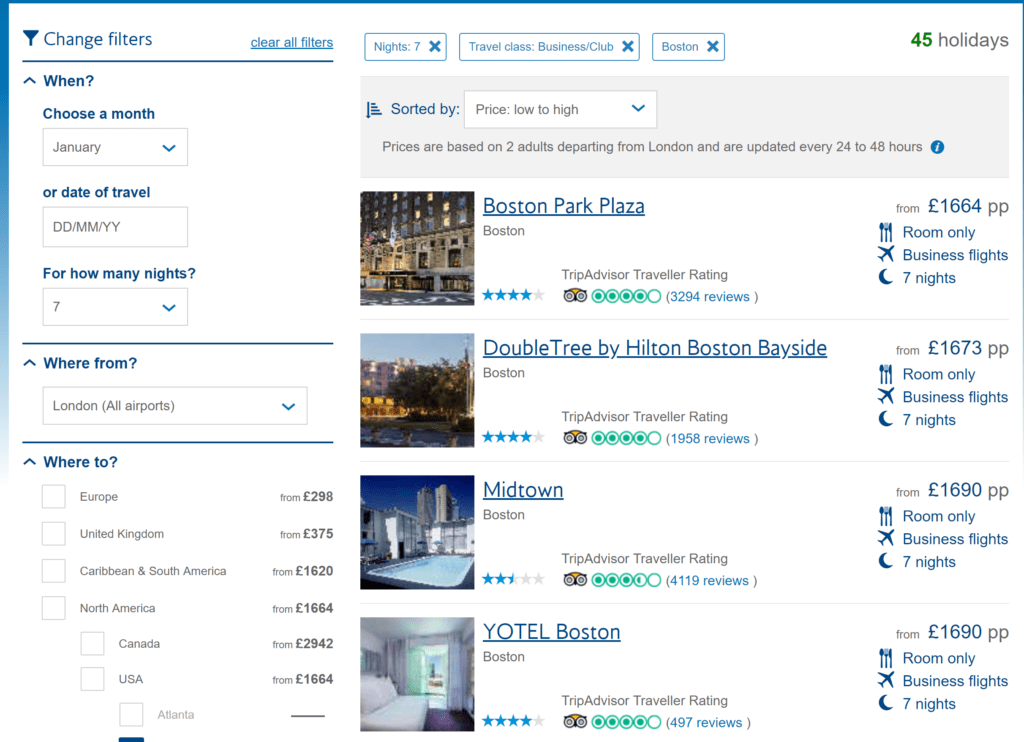This image captures a detailed view of a hotel booking website, specifically focusing on search results for hotels in Boston. Positioned in the top right corner is an option labeled "Change Filters." Below it, under the heading "When," there is an option to "Choose a month," with January selected, or to specify the "Date of Travel," which remains unselected. An additional filter for the duration of stay, "For How Many Nights," is set to 7 nights. 

The departure is noted as "London All Airports" under the "Where From?" section. The "Where To?" section lists numerous destinations including Europe, the United Kingdom, Caribbean, South America, North America, Canada, and the US, with Atlanta specifically mentioned.

Running along the top of the page is a summary bar that states: "Nights: 7, Travel Class: Business/Club, Destination: Boston," and it indicates that there are "45 Holidays" available. Just beneath this, the search results are sorted by "Price, Low to High," with a note that prices are based on two adults departing from London and are updated every 24 to 48 hours.

The search results are visually represented by icons featuring photographs of each hotel. There are four results displayed:

1. **Boston Park Plaza**: The image features a close-up of the hotel's facade. The price listed is "From £1664 PP, Room Only, Business Flights, 7 Nights."
2. **Doubletree by Hilton, Boston Bayside**: This result shows a broader view of the front of the hotel. The price is "From £1673 PP, Room Only, Business Flights, 7 Nights."
3. **Midtown, Boston**: The image highlights a hotel with a pool in the foreground, labeled with a price "From £1690 PP, Room Only, Business Flights, 7 Nights."
4. **Yotel, Boston**: The photograph depicts the interior of a hotel room, also priced "From £1690 PP, Room Only, Business Flights, 7 Nights."